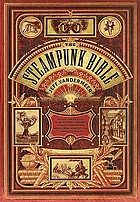The book cover is intricately designed with a generally dark red background framed by a light brown border. The central focal point is a fan-like shape in mostly beige, bearing the title "The Steampunk Bible" in black text. Beneath the title, also arranged in an arc to mimic the fan, is the author’s name, Jeff Vandermeer. At the top of the cover, there are three distinct badges: circular ones on the left and right, and a horizontal rectangle in the center adorned with a black and white depiction resembling goggles or large eyes. Below the fan-like shape, a U-shaped layout features various steampunk-related images. On the left of this U-shape is a vertical picture of a black and white tree, while on the right is an image of a character. At the bottom, there's a scene with several characters, although the details are somewhat illegible. In the center of the cover, a red plaque with small black text adds to the vintage and intricate aesthetic of the design.